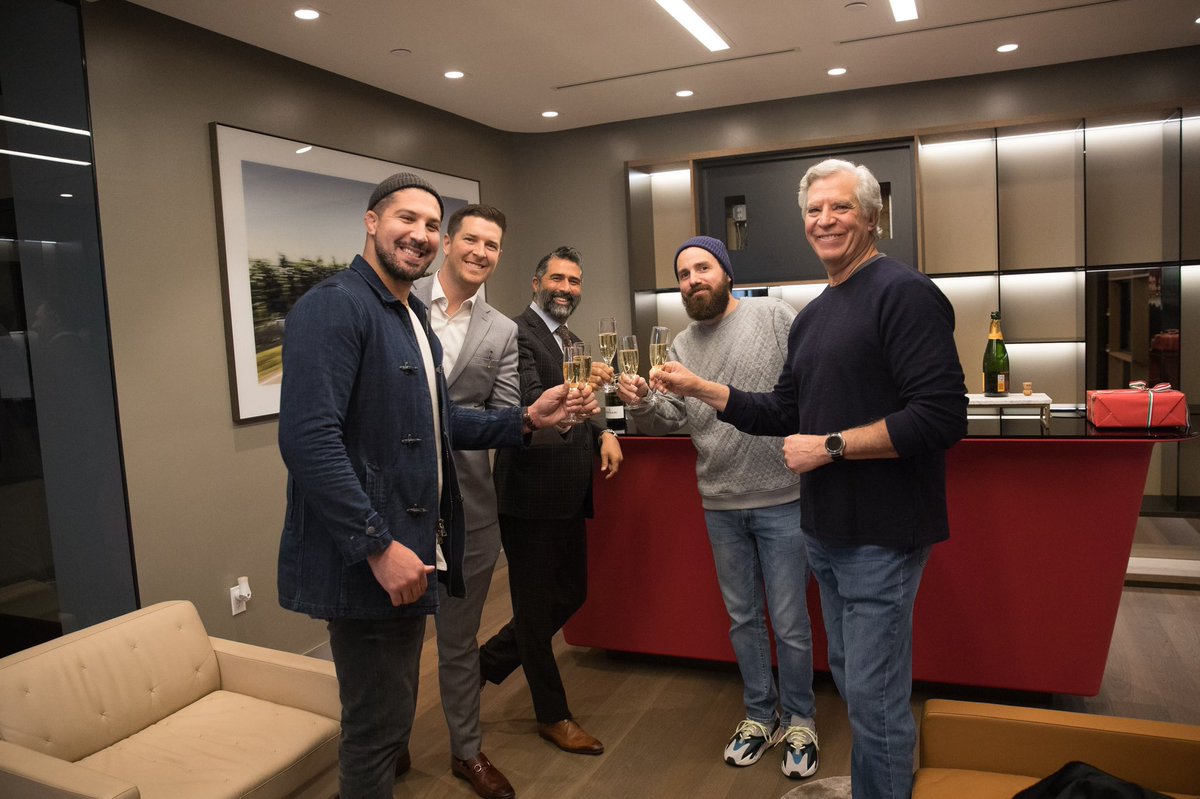The photograph captures a group of five gentlemen standing in what appears to be an apartment or hotel room. They are all holding identical wine glasses and posing for the picture with their glasses raised towards the center, indicating a celebratory or convivial atmosphere. The group is split into three men on the left and two on the right. Their attire ranges from business casual to more formal, with one individual in a full suit and another in a suit without a tie, while the remaining three are dressed more casually. 

Behind them, a bar area can be seen with a wine bottle placed on the counter. The room is furnished with chairs and has shelves adorning the wall behind the men. A framed picture is mounted on the wall to the left, adding a touch of decor to the setting. The overall scene conveys a relaxed yet sophisticated gathering.